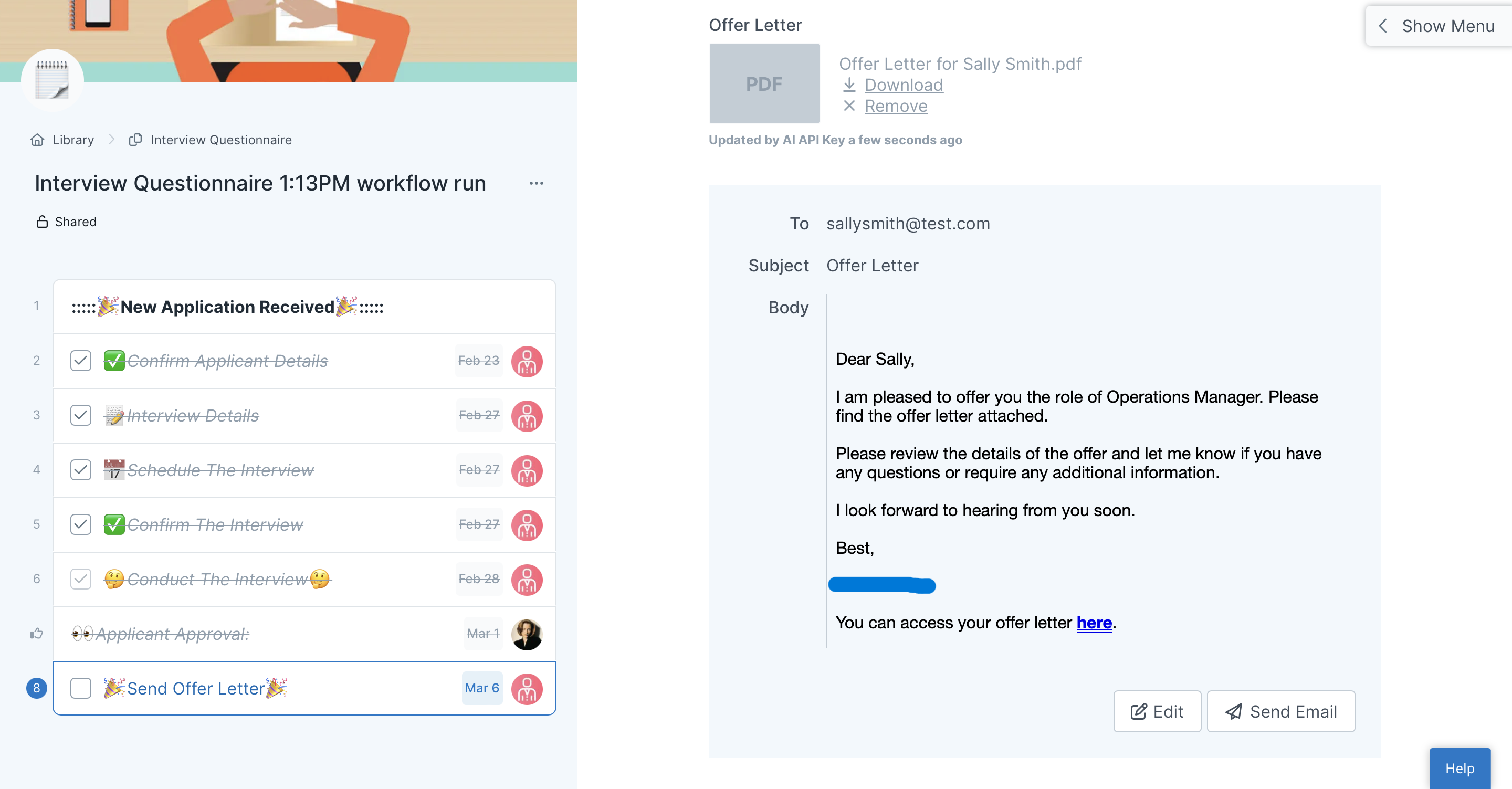The image displayed on a computer screen is divided into two sections. The left side of the screen shows a document titled "Interview Questions," with a timestamp indicating "1:13 p.m. Workflow Run." The document features a cartoonish illustration of an individual sitting at a desk, with their hand placed on a piece of paper labeled "Library." The top of the document reads "Interview Questionnaire," and beneath that, there is a list starting with "New Application Received" followed by sections like "Confirm Applicant Details" and "Interview Details," among others.

On the right side of the screen, there is a document titled "Offer Letter," saved as a PDF named "offer_letter_for_sally_smith.pdf." This section provides options to download or remove the file. The letter is addressed to "sally.smith@test.com" and begins with "Dear Sally," stating, "I am pleased to offer you the role of Operations Manager. Please find the offer letter attached. Please review the details of the offer and let me know if you have any questions or require any additional information. I look forward to hearing from you soon. Best," and concludes with the sender's name, which is obscured with a Sharpie for privacy.